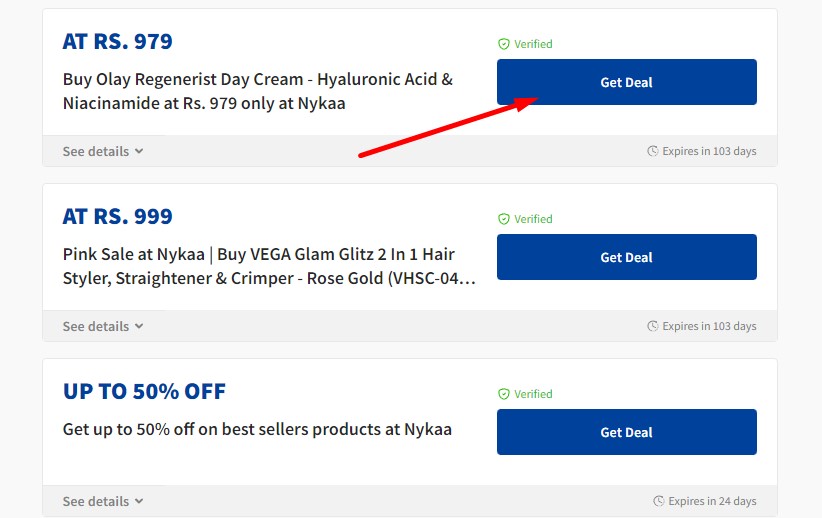A minimalistic website displays three skincare products in a simple, store-like format reminiscent of Amazon but more streamlined. The highlighted item is ATRS.979 Biolay Regenerist Day Cream, which contains Hyaluronic Acid and Niacinamide, priced at RS.979. It's available exclusively at Nykaa (N-Y-K-A-A). Additionally, there are two other skincare products on display. One catchy offer showcases a "Get up to 50% off on bestseller products at Nykaa," with a discount expiring in 24 days.

To the right of each product listing, there is a "Get Deal" button, accompanied by a red arrow pointing at the first button. Each deal is tagged with "verified" to assure legitimacy. The current active deal for the highlighted product expires in 103 days.

The clean design and specific call-to-actions suggest the platform might be a coupon application or Nykaa’s own site offering deals. However, the context of Nykaa is not further explained.